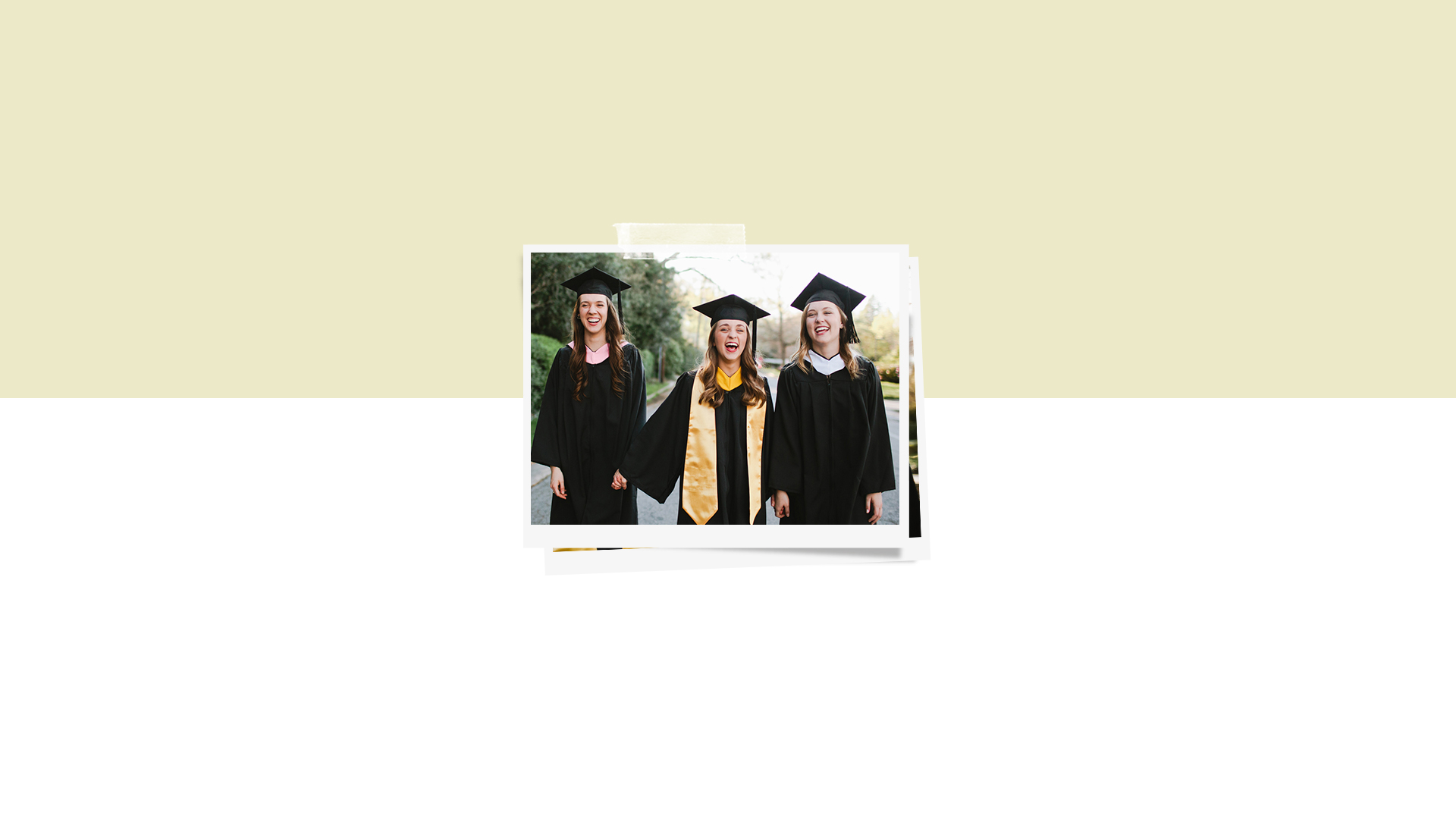The image showcases a nostalgic, Polaroid-inspired scene set against a two-tone backdrop, with a white lower portion and a light beige-green upper portion. Centrally featured are two snapshots, the top one prominently displaying three jubilant female graduates. They are all in traditional black caps and gowns; the two on the outside wear white stoles, while the one in the middle is distinguished by a yellow valedictorian sash and ribbon. They appear to be walking down a sidewalk, holding hands and laughing, with trees lining the background. Their youthful exuberance suggests a high school or college graduation, captured in a moment of shared happiness. The photograph is taped to the backdrop, overlaying another partially visible image, adding to the layered, scrapbook-like aesthetic.